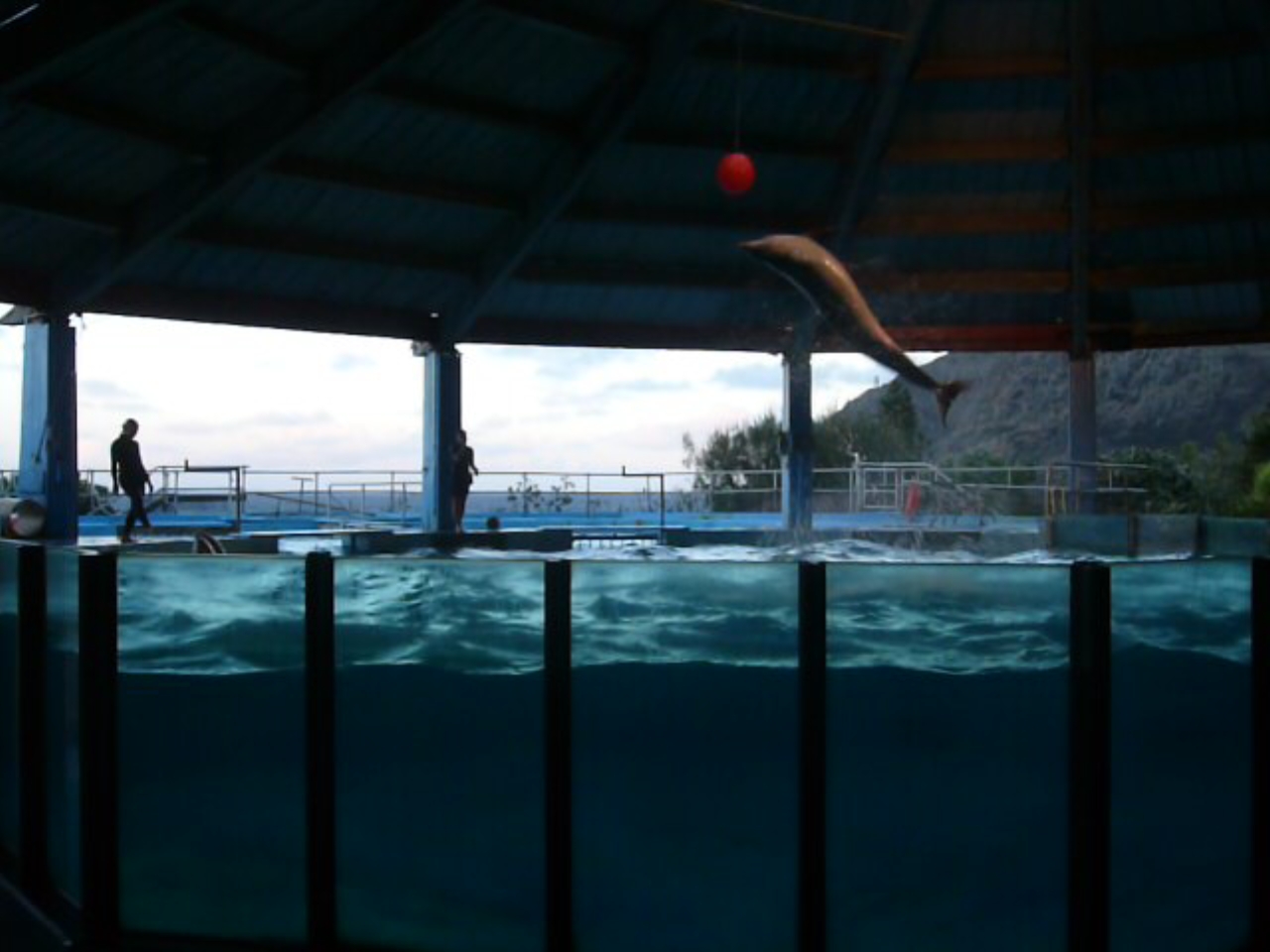The image depicts an open-air aquatic tank, resembling a SeaWorld-type enclosure with a roof but no walls, providing a view of distant mountains and the ocean. The sizable water tank, as large as a small house, has dark blue water and clear plexiglass sides. In the center, slightly to the right, a bronze-statue-like dolphin appears to be jumping toward a red ball suspended above it. To the left, a person in a scuba or wetsuit stands at the water's edge, possibly preparing to enter the tank. Another individual, partially obscured by a pillar, stands to the left of center, likely a dolphin trainer observing the scene. The background features a bright, partially cloudy sky. Concrete bars support the roof structure, adding to the open, airy feel of the space.